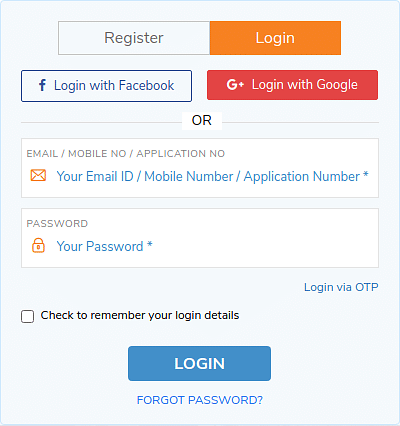Displayed in the image is a mobile application's login page, characterized by a clean, user-friendly interface with a predominantly blue background. At the top, there are two main options: "Register" in green and "Login" in orange. The page also includes social media login options, featuring an orange "Login with Facebook" button and a green and red "Login with Google" button.

Below these options, there are fields to enter your credentials. The first input field is labeled "Email/Mobile Application Number," where users are instructed to type their email address or mobile number. Directly beneath this field is a password input section, identified by an orange lock symbol. The placeholder text in the password field reads "Your Password" in blue, accompanied by an asterisk to indicate it is a required field.

Additional options on the page include a checkbox to "Remember your login details," and an alternative login method labeled "Login via OTP" in blue. Below these options is a prominent blue "Login" button. At the bottom of the login interface, there's a "Forgot Password?" link in all caps.

Overall, this login page facilitates multiple methods for users to access the application, with clear and colorful buttons enhancing navigability.